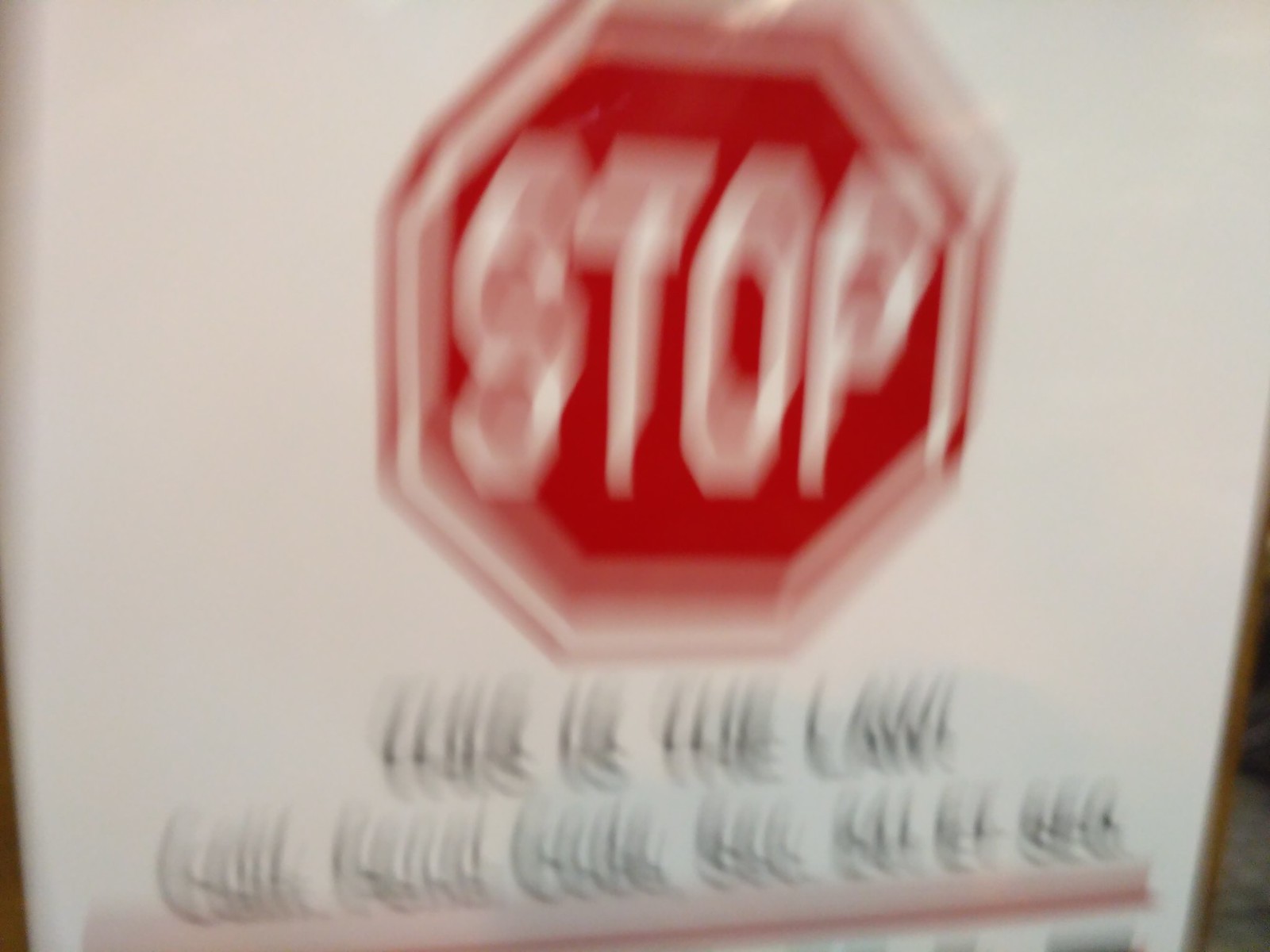A white piece of paper dominates the image, prominently displaying a red, octagonal stop sign in the center. The stop sign features the word "STOP" in bold white text, mirroring the appearance of a traditional red road sign. Above the stop sign, the text reads "This is the law," suggesting a regulatory or warning message. Below the stop sign, additional text alludes to something related to "Code Rec," though it is partially obscured and difficult to read in detail. A red line beneath this text seems to underline and emphasize the message. The overall impression is that this sign is intended for placement in areas where access is restricted, such as on a door in a restaurant or another private space. The stark contrast of the white paper background and the vibrant red stop sign captures the viewer's attention and communicates a clear message to halt or comply with posted instructions.